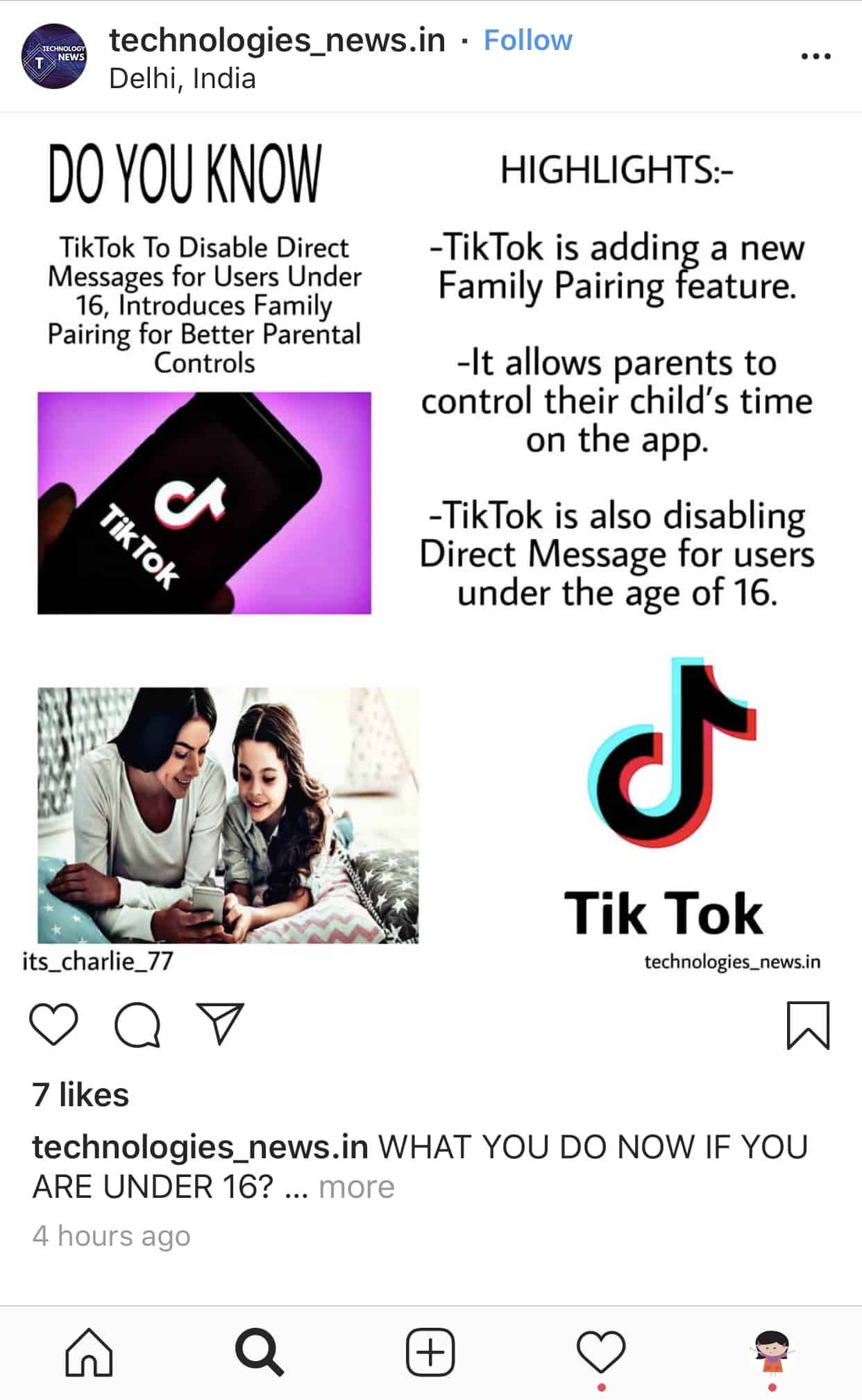### Descriptive Caption:

The image showcases a tweet from the account "technologies_news.IN," which is displayed on the left side against a white background. The account handle and name are displayed in black text, and their location "Delhi, India" is mentioned beneath the username. A blue "Follow" button and a menu icon with three dots are also visible next to the account name.

The tweet discusses TikTok's new updates aimed at improving safety and parental control on the platform. It begins with the intriguing prompt, "Do you know TikTok to disable direct messages for users under 16, introduces Family Pairing for better controls," followed by an image of a smartphone showing the TikTok logo and a stock photo of a mother and daughter presumably using a phone while sitting on a bed.

The tweet is further elaborated upon in the highlights section on the right side, which reads: "TikTok is adding a new Family Pairing feature that allows parents to control their children's time on the app. TikTok is also disabling direct messages for users under 16." The branding is consistent with a small black TikTok logo followed by "TikTok" and the handle repeat "technologies_news.IN."

The tweet has garnered seven likes and poses the question, "What do you do now if you're under 16?" in black text. At the bottom of the tweet interface, standard icons for Home, Search (magnifying glass), Post (a square with a plus sign), Notifications (heart), and Profile (a personal icon) are centrally displayed.